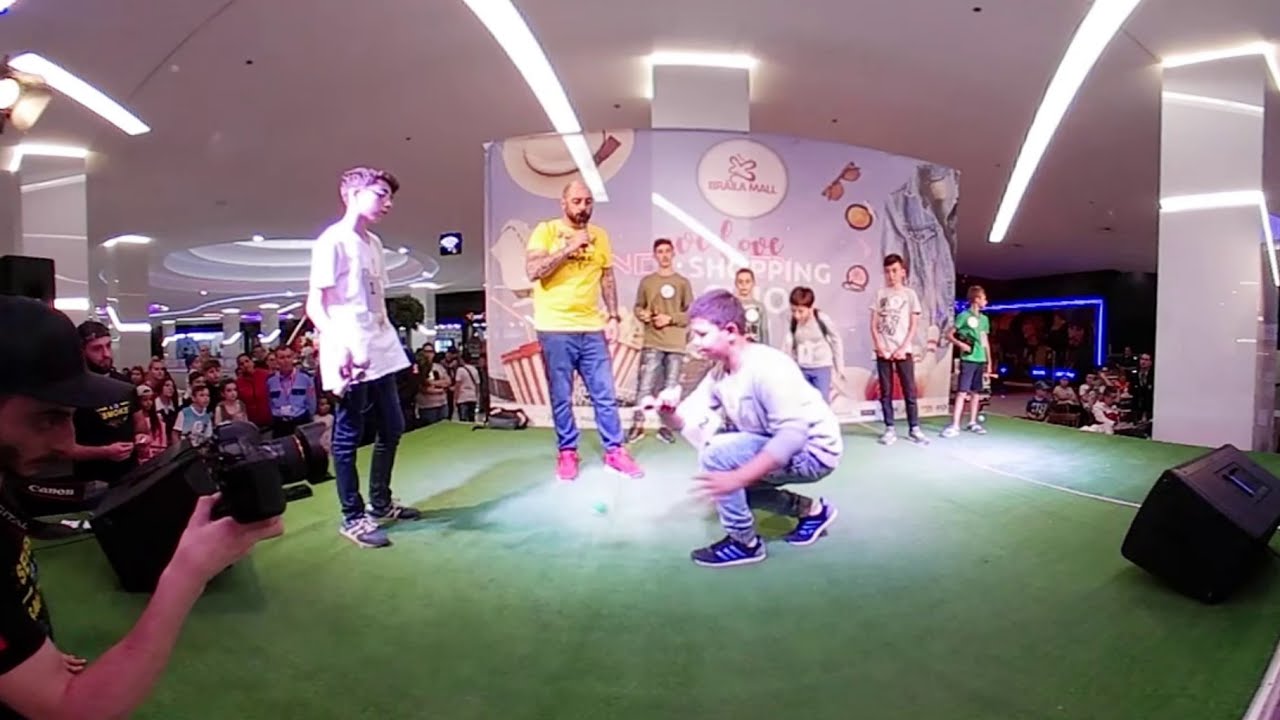In this vibrant indoor scene, a dynamic performance unfolds on a stage with a distinct green floor. Central to the stage, a boy with seemingly purple-tinted hair, due to the striking light, is crouched down, facing left. He sports sneakers with blue stripes and is observed keenly by other children, one of whom wears glasses and a dark, baggy t-shirt. Another prominent figure on the stage is a man dressed in a yellow short-sleeve t-shirt, blue jeans, and striking reddish-pink sneakers. He appears to be speaking into a microphone, perhaps orchestrating the event. 

Behind them, a large, colorful sign boldly displays "Love Shopping," adorned with images of sunglasses, hats, and other items. Adding to the scene's bustle, a person with a camera or spotlight, identifiable by their black hat and positioned in the left bottom corner, is capturing the event. The background hints at an indoor mall environment, with spectators and families gathered to watch the performance, illuminated by white strip and circular lighting from the ceiling. Seven children, possibly competitors, are also visible, suggesting an organized competition or school performance.